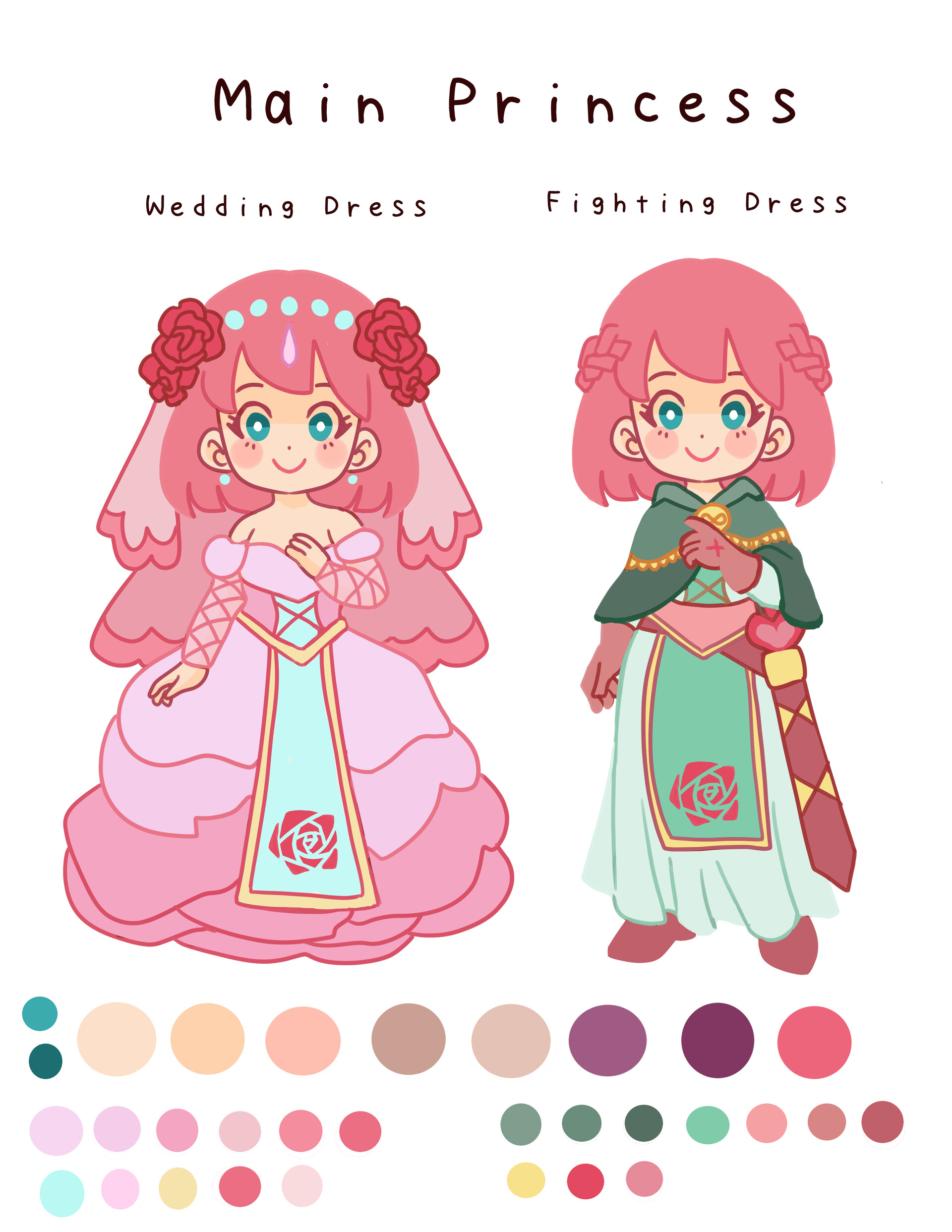The image is a detailed cartoon featuring a female character named "Main Princess Center" against a solid white background. At the top, the text reads "There's No Border Around It." The character is depicted in two distinct outfits: on the left, she wears a pink wedding dress adorned with red roses on each side of her veil, and on the right, she sports a fighting dress consisting of a light green, long flowing gown with a green wrap around her chest and a sword with pink and gold details attached to her hip. She retains her pink hairstyle in both outfits. The character's left hand is gently placed on her chest in both poses. Below each outfit, there are small colored circles, presumably for selecting different color schemes for the character. The image is richly colored with a palette that includes shades of teal, mint green, light blue, violet, brown, beige, tan, coral, various pinks, yellow, pastel yellow, and peach. The style of the artwork suggests it could be a drawing, a painting, or a digital creation.